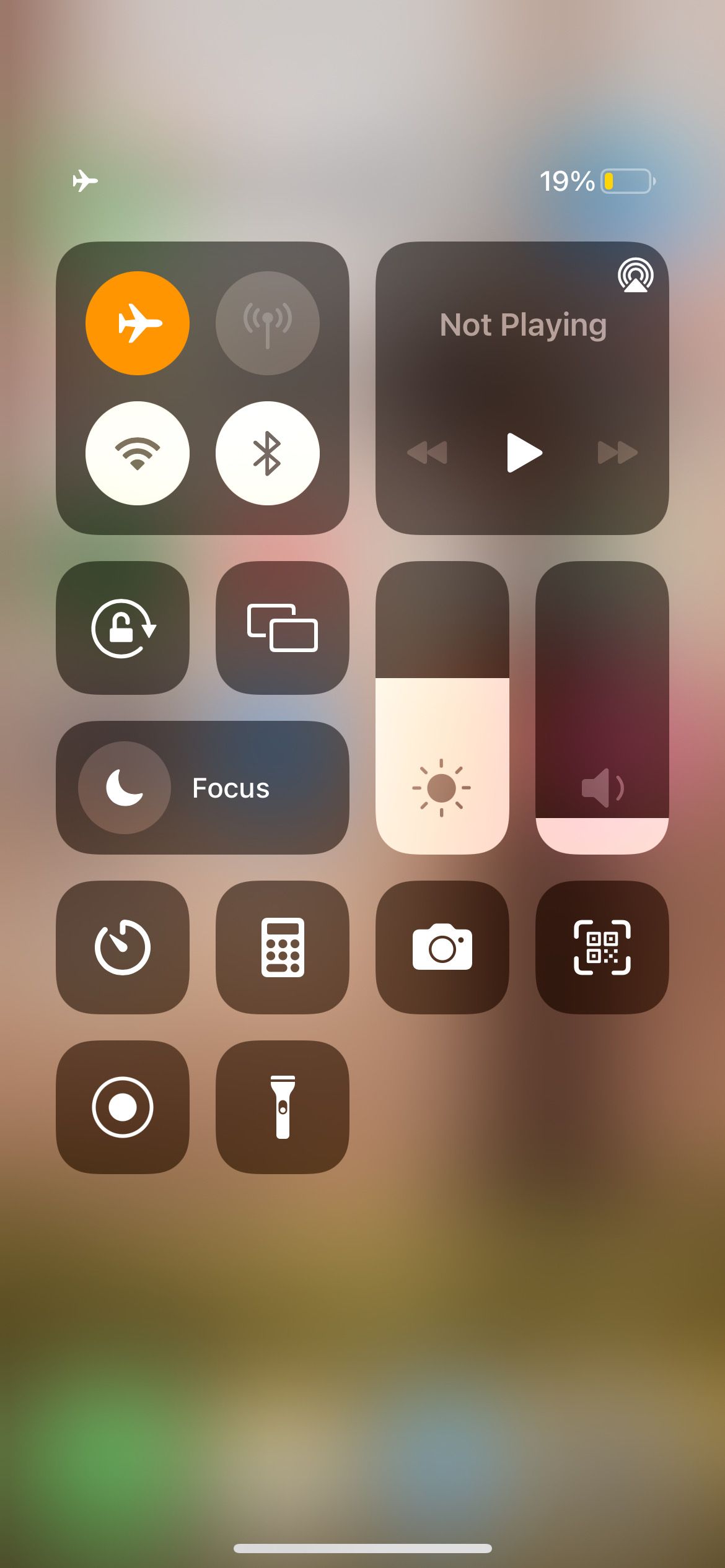The screenshot displays a smartphone's settings menu oriented in portrait mode. The settings interface, accessed by swiping down from the top of the screen twice, shows the various active features. In the top left corner, an orange airplane mode icon indicates it is enabled. Directly below, illuminated icons for Wi-Fi and Bluetooth show that both are active while a disabled mobile data icon sits at the top right. The upper right section also shows "Not playing," indicating no current media playback. Below these indicators, the brightness level is set a little above halfway, and the sound volume is almost at its minimum. Lastly, the top right corner displays the battery percentage at a critical 19%.